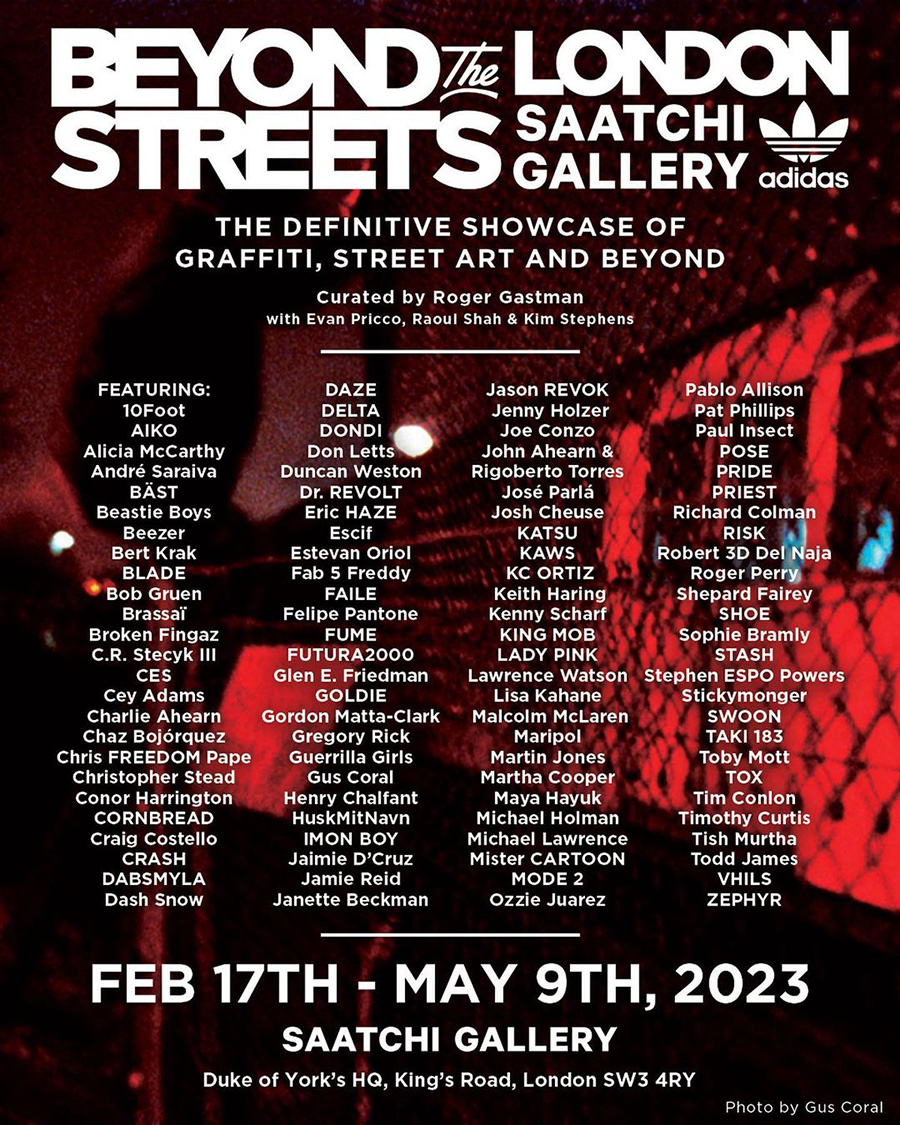The image is a vibrant promotional poster for "Beyond the Streets of London" at the Saatchi Gallery, meticulously detailed with a red background featuring a chain link fence and a figure climbing it. Presented by Adidas, whose logo is prominently displayed, the poster is adorned with white text. At the top, it boldly states: "Beyond the Streets of London at the Saatchi Gallery, the Definitive Showcase of Graffiti, Street Art, and Beyond." This exhibit, running from February 17th through May 19th, 2023, is curated by Roger Gassman, with contributions from Evan Prigoth, Raul Sal, and Kim Stephens. It showcases works from numerous artists, including Ten Foot, Akio, Alicia McCarthy, Andre Sarria, Bast, Beastie Boys, Beezer, Burk Crack, Blade, Rogue-One, Broken Fingers, C.R. Stecyk III, Siss, C.K. Adams, Charlie Ahearn, Chaz Bojorquez, Chris 'Freedom' Pape, Christopher 'Daze' Ellis, Connor Harrington, Cornbread, Craig Costello, Crash, Dondi, Don Letts, Donde, Dr. Revolt, Eric Haze, Eroné, Estevan Oriol, Fab 5 Freddy, Vhils, Felipe Pantone, Fumero, and Futura 2000. The location details are clearly listed at the bottom: "Saatchi Gallery, Duke of York's HQ, King's Road, London, SW3 4RY," and the photo credit is attributed to Gus Corral in the bottom right corner.